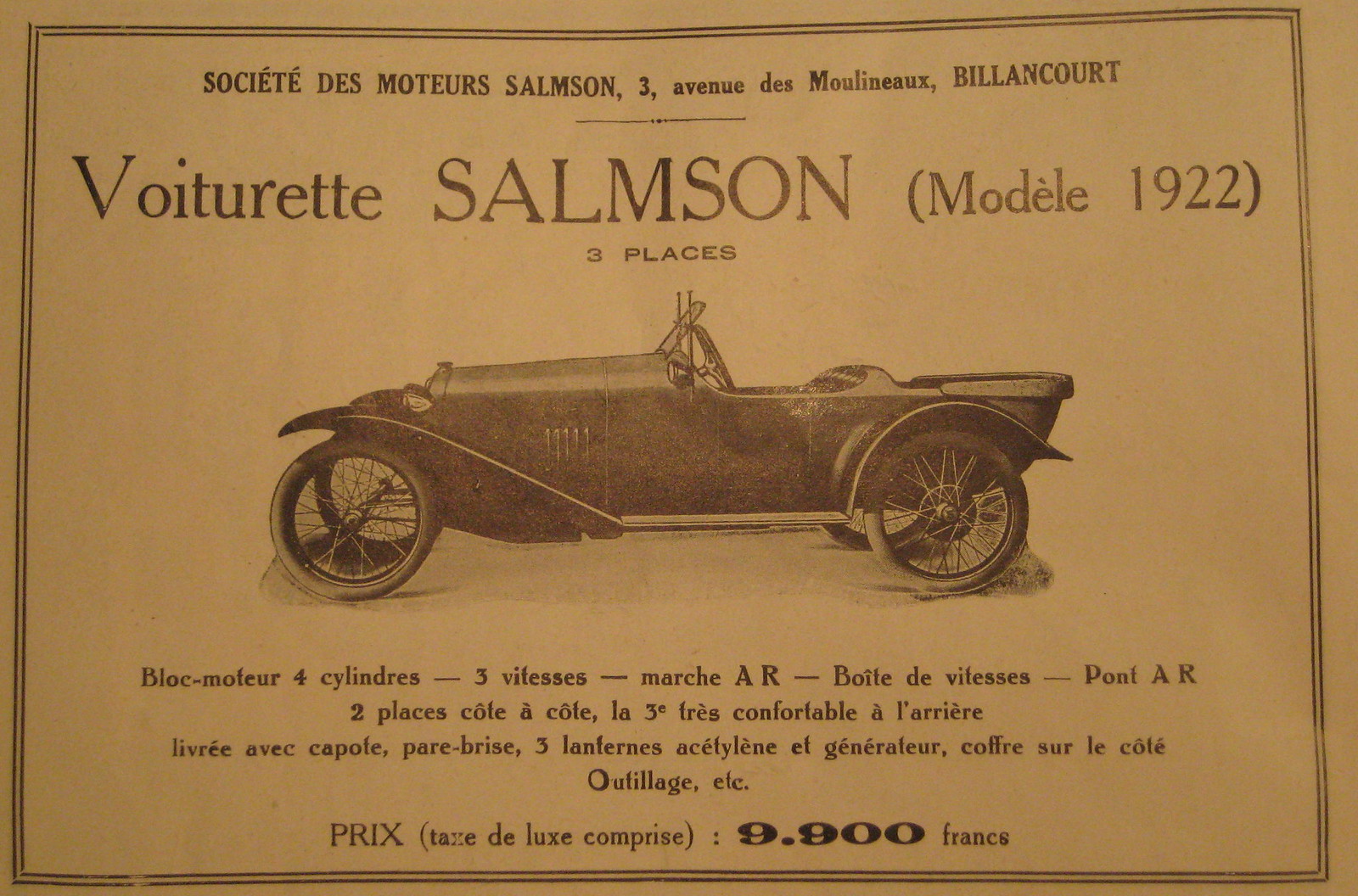This antique advertisement, likely from a French magazine or newspaper, is a rectangular black and white image with a double black-lined border. The paper has a brownish or tan hue, possibly due to lighting or age. The text, written entirely in French, begins at the top with "Société des Moteurs Salmson, 3 Avenue des Monceau, Billancourt," indicating the company's Paris location. The advertisement features a "Vaux-Tourette Samson Model 1922," with a prominent vintage car image at its center. The car is an open-top convertible with a long hood, four large bicycle-style spoke wheels, a prominent front and back fender, two front seats, and possibly two smaller rear seats. It features a short windshield and a small steering wheel, characteristic of early 1920s design. Below the image, detailed specifications in French highlight the car's four-cylinder engine and other attributes. At the bottom, the price is listed as "PRIX 9.900 francs."